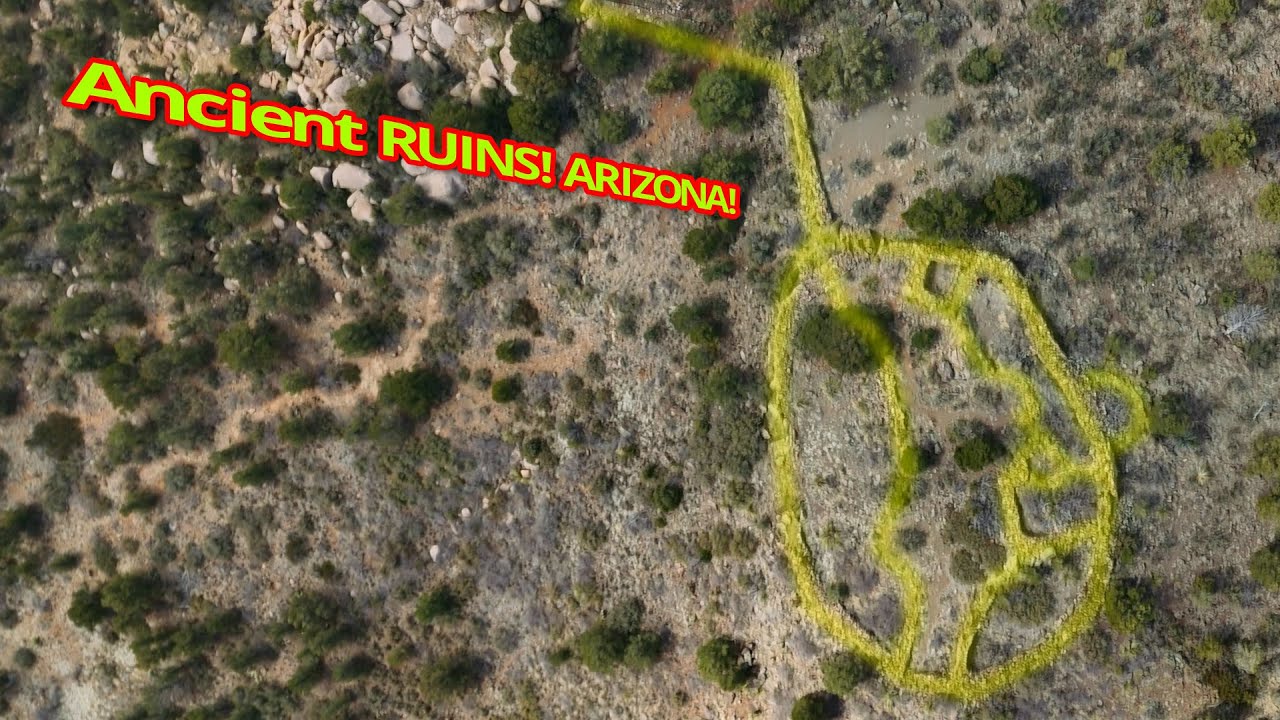The image captures an aerial, bird's-eye view of a desert terrain in Arizona, presented in muted tones of dusty brown and gray interspersed with scattered dark green bushes and shrubs. A significant portion of the photo is marked with a large yellow outlined circle, reminiscent of a turtle shell, featuring squiggly lines and extending with a long yellow line. This marking indicates areas of interest, possibly ancient ruins. In the upper left corner of the photograph, text in neon yellow with a red outline prominently reads "Ancient Ruins Arizona!" The terrain is typical of an arid desert with large chunky white stones to the left and a barren, sand-covered landscape. The entire scene lacks any visible people or animals but features a variety of vegetation and rocks of various sizes.